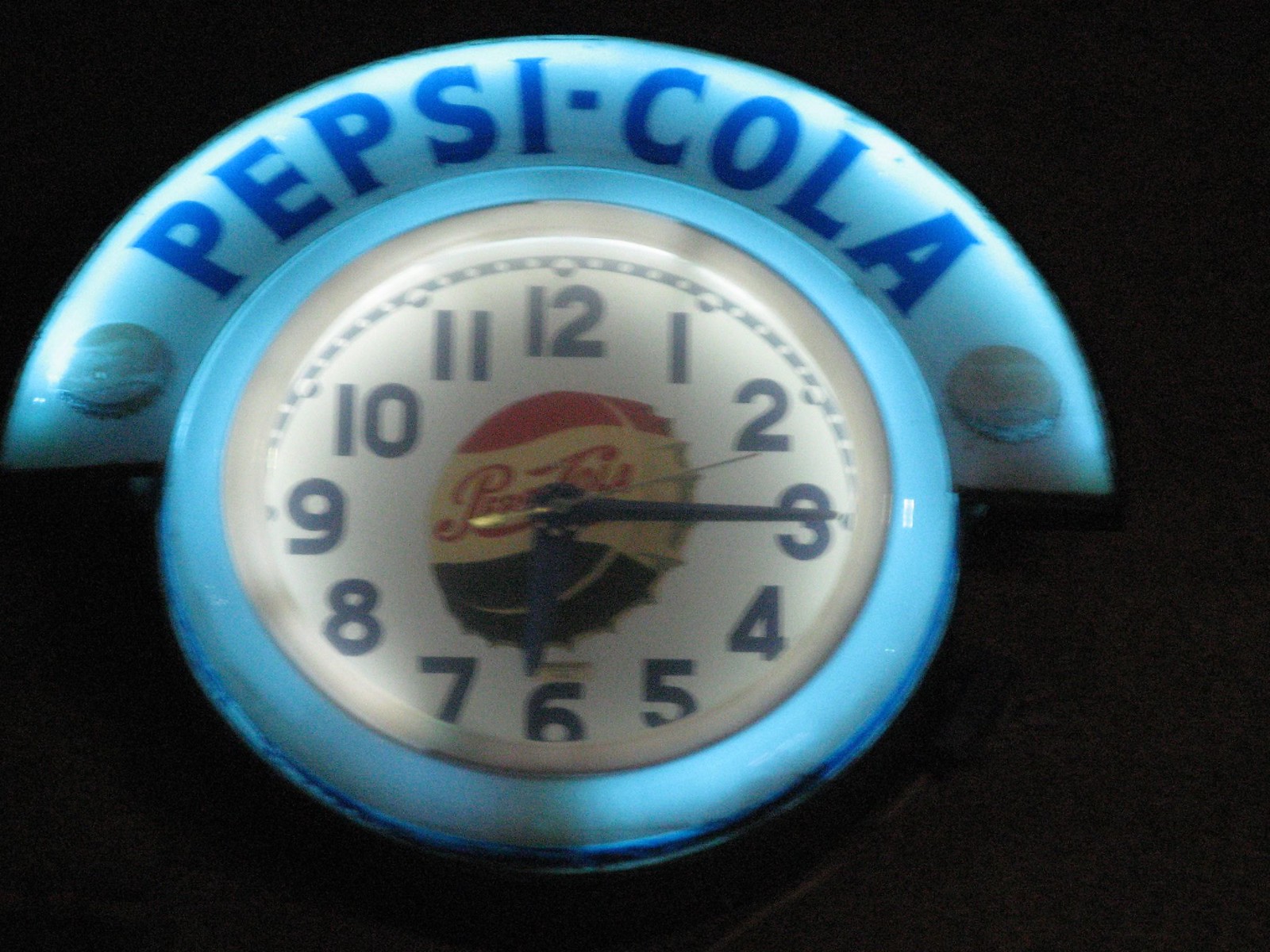This image depicts a vintage Pepsi-Cola wall clock, likely used for advertising in a grocery store or restaurant. The clock has a backlit, bright blue border and a predominantly white face with bold, dark blue numbers clearly indicating the time as 6:15. The clock's dark blue hour and minute hands and a barely visible gold second hand are set against the white background. At the center of the clock face, there is a vintage-style Pepsi-Cola bottle cap, displaying the brand's classic red, white, and blue color scheme with the Pepsi-Cola logo. Above the round clock face, there's a wide, semi-circular, blue-edged extension bearing the Pepsi-Cola name in dark blue letters. The entire background of the image is black, which emphasizes the illuminated clock and its distinct Pepsi branding, including a dark blue dashed line outlining the top half of the clock.